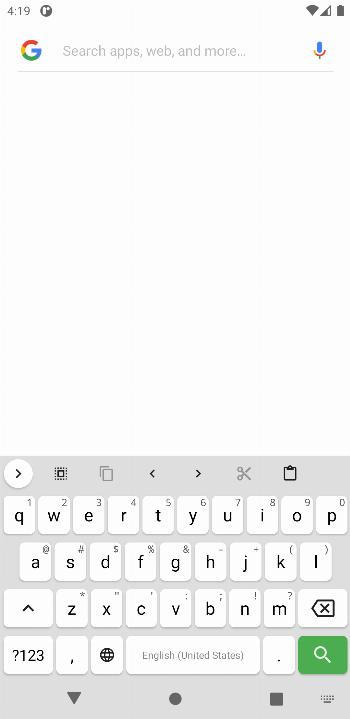The image appears to be a screenshot of a smartphone keyboard interface. 

Starting from the bottom of the image, there is a gray keyboard layout. In the bottom left corner, a white circle with an arrow pointing to the right is visible. Moving upwards, the keys on the keyboard are predominantly white with different letters, symbols, and numbers marked in black.

The first row of keys from left to right features the letters: Q, W, E, R, T, Y, U, I, O, P. The upper right-hand corner of this row is labeled with the numbers: 1, 2, 3, 4, 5, 6, 7, 8, 9, 0.

In the second row, the keys display the letters: A, S, D, F, G, H, J, K, L. Additional symbols are present in the corners of these keys, including the at symbol (@), pound sign (#), dollar sign ($), percentage (%), dash, underscore (_), open parentheses "(", and close parentheses ")".

The third row includes the letters: Z, X, C, V, B, N, M, along with a backspace key depicted as an arrow with an "X" in it. Additional symbols in this row include a star (*), single and double quotation marks ("), semicolon (;), exclamation point (!), and question mark (?).

Beneath these rows is an assortment of special function keys: a series of numbers: 1, 2, 3, 4, with a question mark (?), comma (,), a black globe icon, a space bar labeled "English, United States," a period (.), and finally, a green key with a white magnifying glass icon.